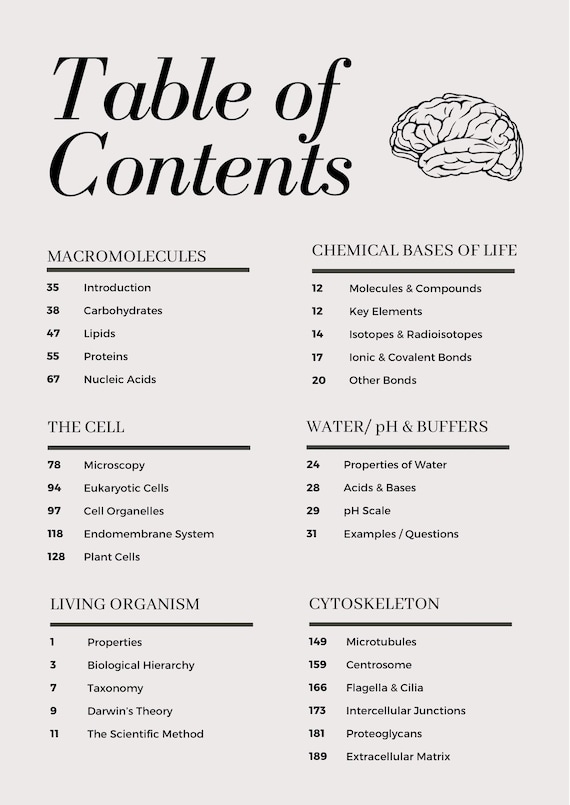The image depicts a black-and-white page from a book, prominently titled "Table of Contents" at the top left. Opposite this title, on the top right, is an intricate illustration of a human brain in black ink. Below the heading, the page is divided into six main sections, each with a comprehensive list of subsections and corresponding page numbers. 

The first section, titled "Macromolecules," begins with an "Introduction" (pg. 35), followed by "Carbohydrates" (pg. 38), "Lipids" (pg. 47), "Proteins" (pg. 55), and "Nucleic Acids" (pg. 67). The second section, "The Cell," includes topics such as "Microscopy" (pg. 78), "Eukaryotic Cells" (pg. 94), "Cell Organelles," "Endomembrane System," and "Plant Cells." 

Following this, the "Living Organisms" section covers "Properties," "Biological Hierarchy," "Taxonomy," "Darwin's Theory," and "The Scientific Method." The "Chemical Bases of Life" section delves into "Molecules and Compounds," "Key Elements," "Isotopes and Radioisotopes," "Ionic and Covalent Bonds," and "Other Bonds."

Next, the "Water/pH and Buffers" section discusses "Properties of Water" (pg. 24), "Acids and Bases" (pg. 28), "pH Scale" (pg. 29), and includes "Examples and Questions" (pg. 31). Finally, the "Cytoskeleton" section is broken down into "Microtubules" (pg. 149), "Centrosome" (pg. 159), "Flagella and Cilia" (pg. 166), "Intercellular Junctions" (pg. 173), "Proteoglycans" (pg. 181), and "Extracellular Matrix" (pg. 189).

The structured layout and detailed subsections offer a thorough overview of the book’s content, essential for anyone studying these topics.